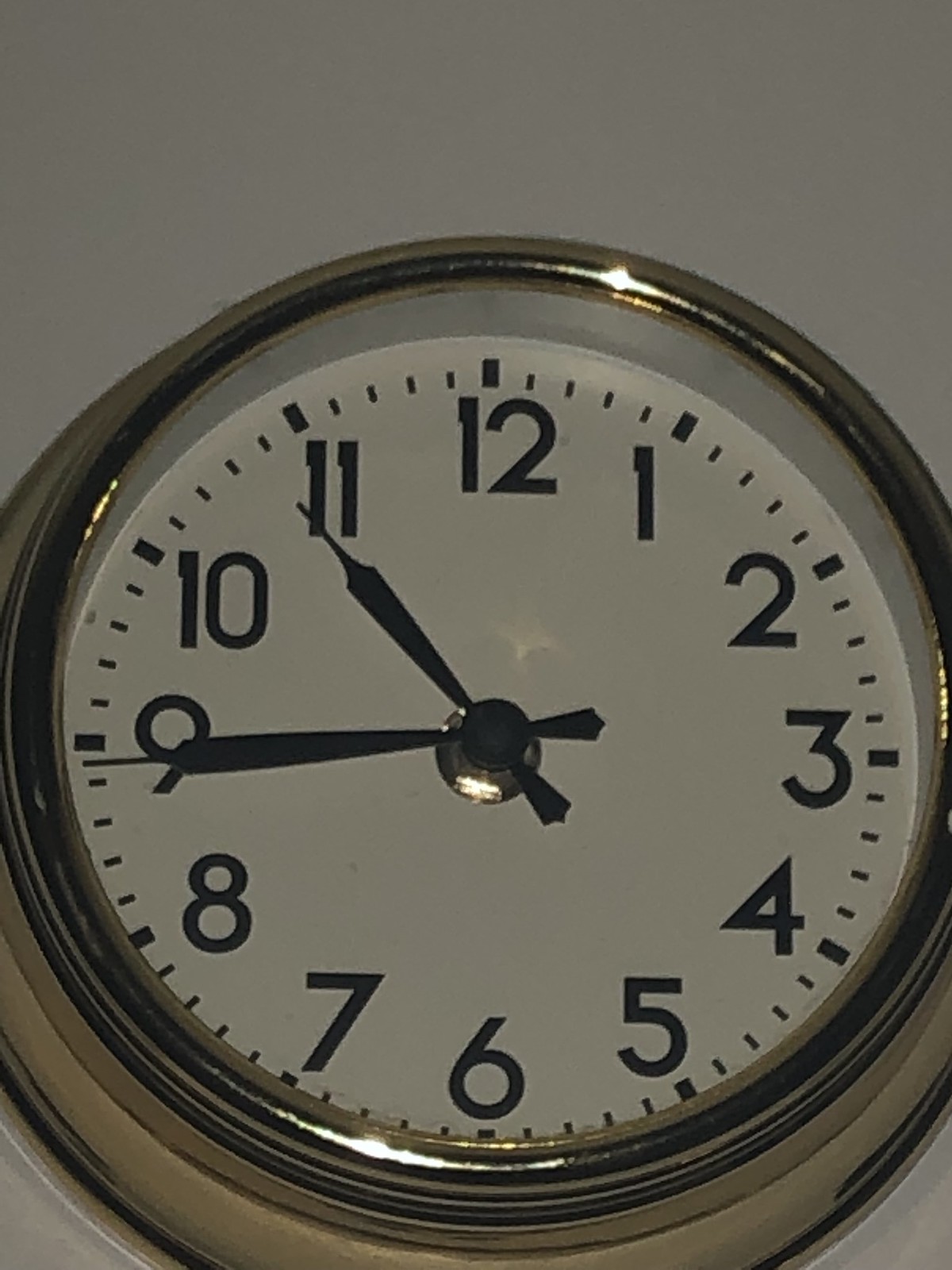In a dimly lit room, a round clock adorns the wall, showcasing a striking gold exterior. The gold case, textured with multiple layers around its circumference, catches the light with a subtle shine. The clock face is a pristine white, contrasting against the stark black of the numerals and tick marks. The black hands of the clock converge at a central point, anchored by a gold centerpiece that matches the border. The minute hand points just beneath the tick for 9, while the hour hand rests under the tick for 11, indicating the time is nearly 11 o'clock. The design features prominent, pointy ticks at each hour, with four smaller ticks between each. The numerals are simple, standard Arabic digits, enhancing the clock's elegant and classic appearance.